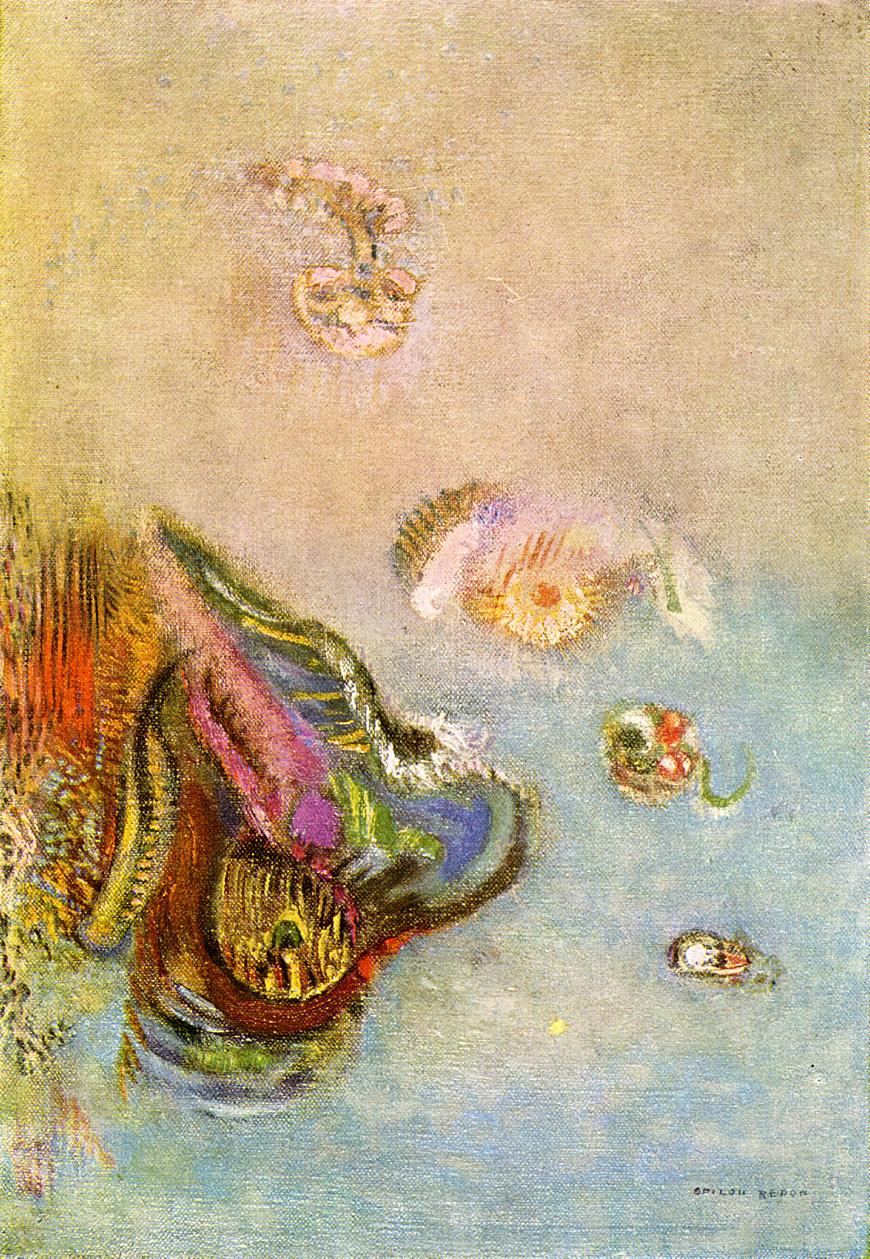This abstract painting features a predominantly blue lower half, suggestive of water, and a sandy beige upper half, reminiscent of a beach. The artwork is replete with vibrant, densely layered brushstrokes, enhancing the texture of the canvas and lending a distinctive impressionistic quality. The centerpiece is a red structure in the lower right quadrant, emerging from a gray tube at the bottom. This structure sports a circular yellow opening with a green middle hole, topped with a pink horn entwined with green ribbons. It is flanked by flame-like orange and yellow shapes.

Above, the sandy beige area hosts a beige and white object at the water's edge, possibly representing a seashell. Adjacent to it is a pink and tan object, adding to the beach-like appearance. To the left, a colorful abstract mass stretches from mid-canvas toward the bottom, incorporating streaks of blue, pink, purple, white, black, green, maroon, and yellow accents, but devoid of definite shapes, enhancing its abstract nature. Floating within the blue area are other colorful objects, including a green, white, and red shape with what appears to be a little green tail, and a smaller black, red, and white entity, each contributing to the dynamic composition of this enigmatic and richly detailed artwork.